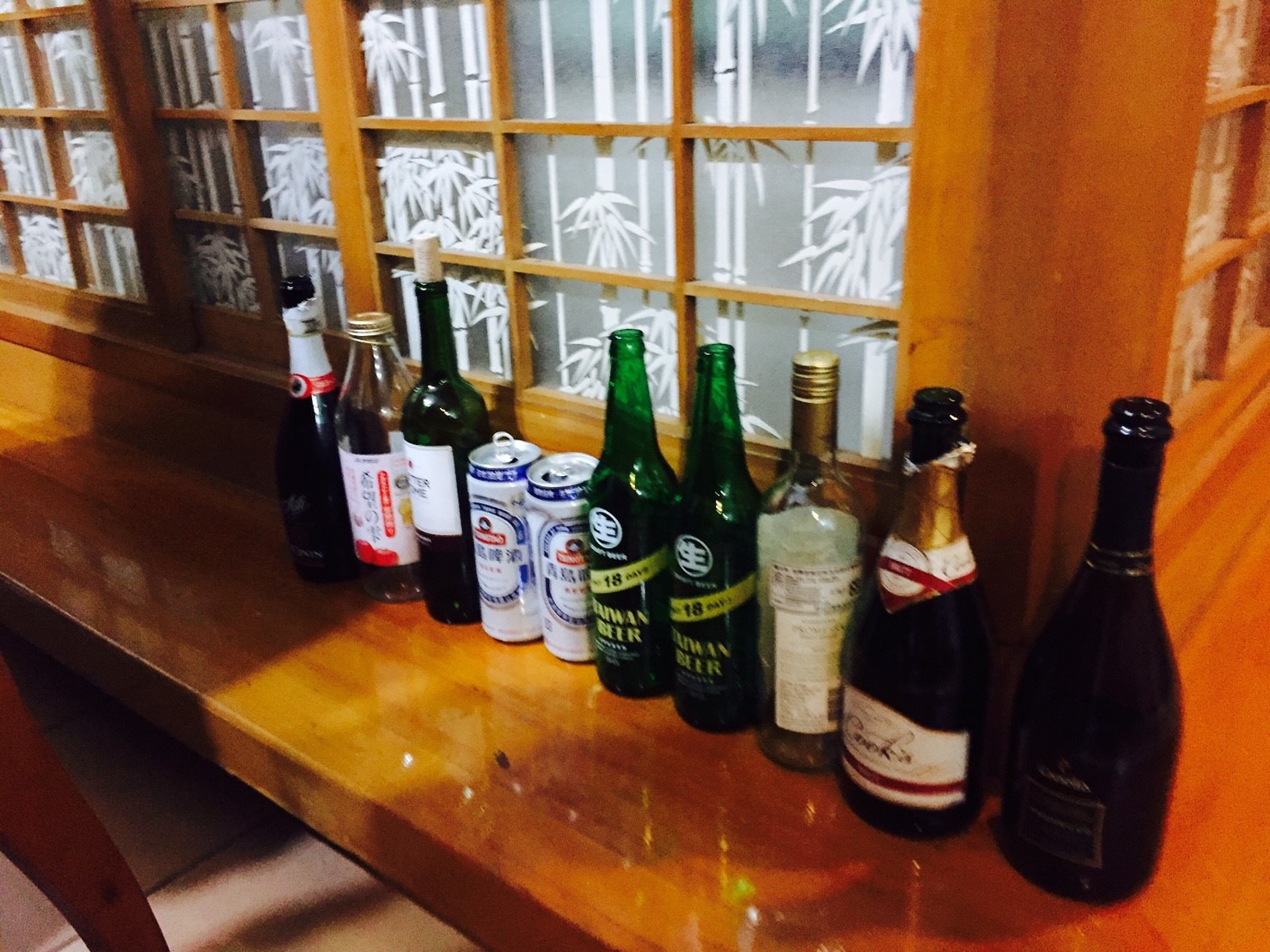The image captures a detailed interior view of a bar, featuring a polished, golden brown wooden counter lined with various bottles and cans of alcoholic drinks. The counter is positioned against a window pane framed with brown wood, intricately etched with white palm trees that add a decorative flair. The bar counter, resembling a half-table or ledge, curves to the right and is used by patrons to enjoy their drinks, with a visible bar stool leg on the left side. The bottles and cans on the counter include a range of beverages: dark brown and champagne-like bottles with labels including "Cooks," clear bottles with gold tops, green beer bottles with oriental lettering and the number '18' in yellow, and opened white cans with red, white, and blue lettering, one of which is noticeably squished. Each bottle varies in color and label design, contributing to the eclectic array of half-empty or empty alcoholic beverages displayed against the backdrop of the elegantly frosted palm tree windows.